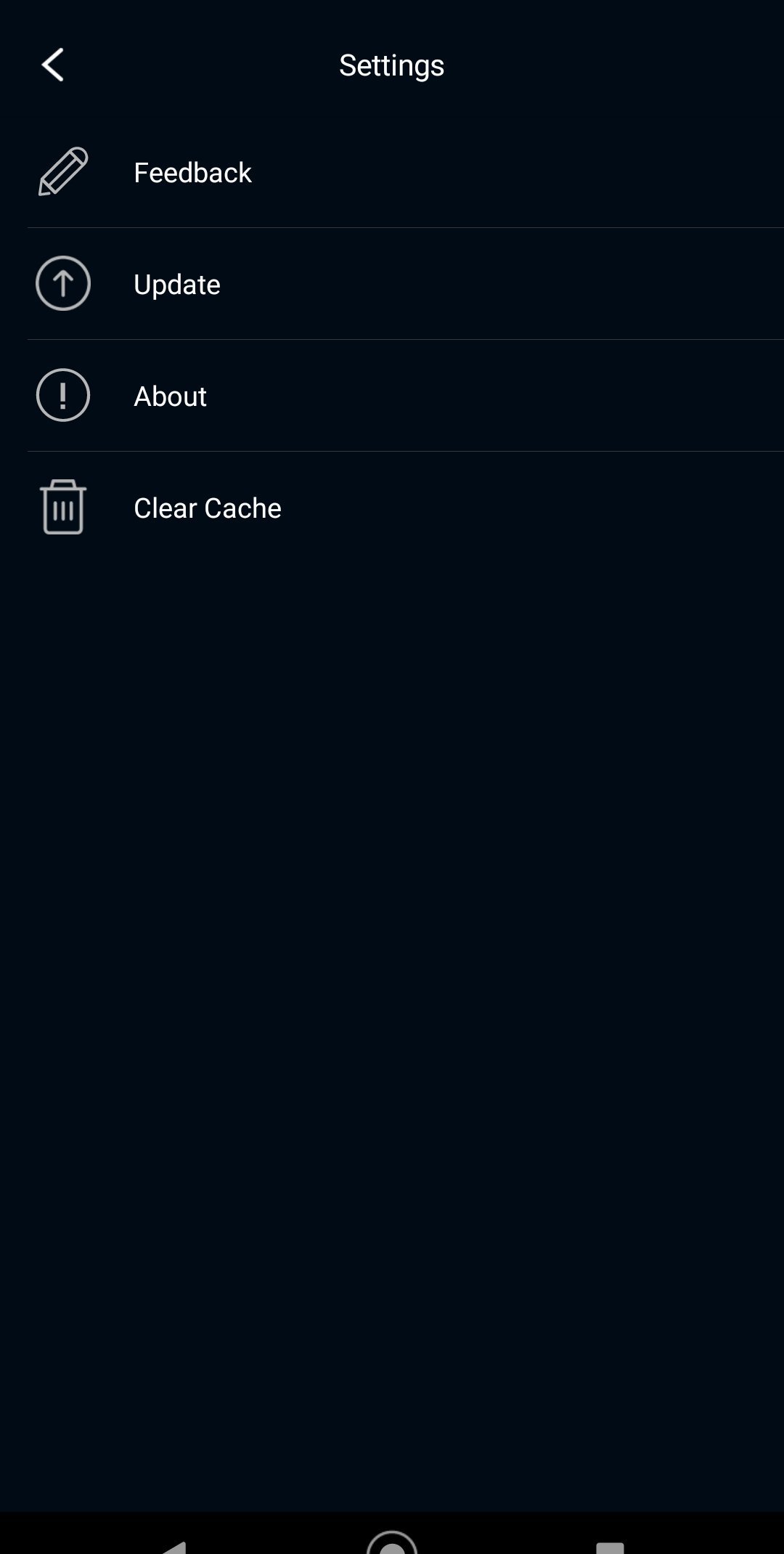The image features a dark blue gradient background that transitions to black towards the top. On the left side, there are navigation options in white text and symbols, including "Settings" accompanied by an arrow pointing to the left. Below, "Feedback" is indicated with a pencil icon, and "Update" is paired with a circular arrow pointing upwards. There is also an "About" section highlighted with an information symbol inside a circle, and "Clear Cache" marked with a trash can icon. At the bottom of the screen, a black rectangle contains partially visible gray icons: a triangle pointing to the left, a circle, and a square.